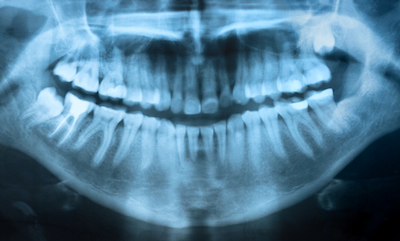This detailed caption describes a panoramic dental x-ray image: 

The x-ray captures a comprehensive view of an individual's mouth, showcasing a clear, albeit slightly blurry, depiction of both the upper and lower teeth along with their roots embedded in the gums. The image predominantly highlights the bony structures, including the front and sides of the jaw, as well as the cheekbones and chin. The teeth are well-aligned, with a small gap visible due to the person's slightly open mouth, which gives a faint smile-like appearance. Notably, the x-ray exhibits a wisdom tooth positioned high and not fully descended on the top right, while the rest of the teeth appear fully erupted and straight. The pale blue hues of the x-ray contrast against the primarily white background, offering a glimpse of some soft tissues and possibly a bit of the shoulder bone, though the focus remains on the dental anatomy. There may be a presence of fillings and a mix of baby and adult teeth, particularly where they overlap. Additionally, the x-ray faintly shows parts of the sinuses, providing a full side-to-side, slightly flattened panoramic view of the dental and jaw structure.